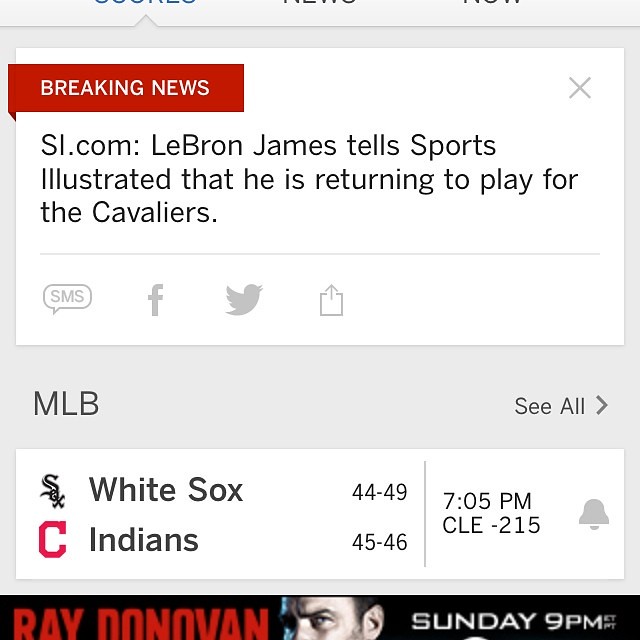The image is a detailed screenshot of a digital news panel. At the top left, "Breaking News" is prominently displayed in red font, followed by text that reads "SI.com." The main headline announces that LeBron James has told Sports Illustrated he is returning to play for the Cavaliers. Below this news brief are icons for sharing on SMS, Facebook, and Twitter. Further down, there's an MLB panel showcasing the matchup between the White Sox and the Indians, with their respective records of 44-49 and 45-46. Additional details include the game time, listed as 7:05 p.m. in Cleveland, and a notation of Cleveland -215. The screen also features logos for both teams. At the very bottom of the screen, there is an advertisement banner for the show "Ray Donovan," which airs on Sunday at 9 p.m. Eastern Time. The entire panel appears to have a gray background, consistent with a mobile app interface. A bell icon is visible in the bottom right corner, along with a partially cut-off "See All" button and other logo buttons at the top of the screen.